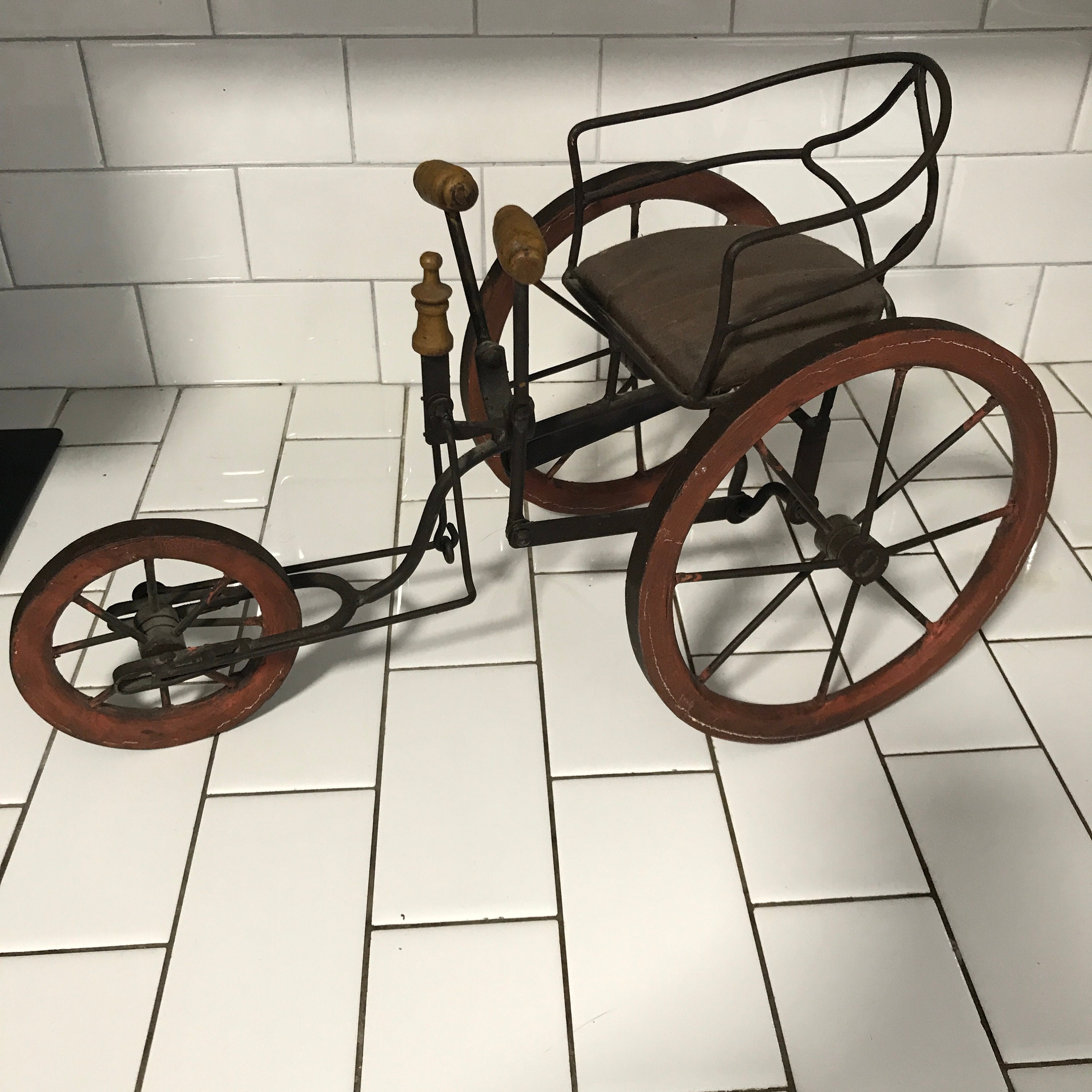This detailed image captures an old-fashioned wheelchair-like contraption, possibly displayed in a museum. The centerpiece of the image is a device that combines elements of a wheelchair and a tricycle. It features two large wooden wheels at the rear and a smaller wooden wheel at the front, highlighting its vintage design. This unique apparatus has a metal chair positioned between the two large rear wheels, equipped with a small cushion for seating comfort. The design includes a pair of handles and a singular stick for steering the front wheel left or right, resembling a tricycle's maneuverability. Additionally, there are two sticks that function similarly to bike pedals, allowing the user to control the movement of the rear wheels. The color palette of the image includes shades of brown, white, black, and a yellowish hue, contributing to the antique appearance of the object. Although there is no text in the image, the intricate details and wooden construction of the wheels underline its historical and possibly museum exhibit setting.